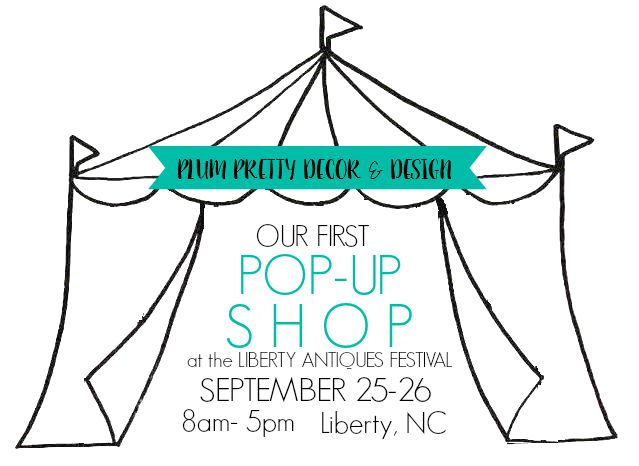This is a black-and-white pencil sketch of a circus-style tent used in an art advertisement for an antiques festival. The tent peaks in the middle and has open curtains at the front, revealing the text inside. It features three flags – one at the top and one on each corner, all pointing to the right. A turquoise-green banner stretches across the top of the tent with the text "Plum Pretty Decor and Design" in black lettering. Beneath the banner, within the open curtains, the text reads: "Our First Pop-Up Shop at the Liberty Antiques Festival, September 25-26, 8 a.m. to 5 p.m., Liberty, North Carolina." This advertisement invites viewers to the event with its artistic and detailed rendering of a classic circus tent.